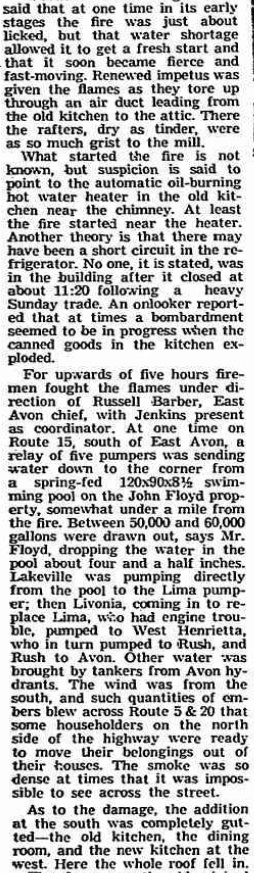This image displays an older black-and-white newspaper column, presenting detailed text organized into indented paragraphs. This column appears to have been photocopied, suggested by a black streak running down the top right-hand side. The text reports on a fire incident, describing that at one point the fire was nearly controlled, but a water shortage allowed it to reignite fiercely. The fire rapidly escalated as it traveled through an air duct leading from an old kitchen to the attic, where dry rafters fueled the flames. While the exact cause of the fire remains unknown, suspicion points to an automatic oil-burning hot water heater near the chimney or possibly a short circuit in the refrigerator.

An eyewitness reported explosions as canned goods in the kitchen burst from the heat. Firemen, directed by East Avon Chief Russell Barber with Jenkins as coordinator, battled the blaze for over five hours. A relay of five pumpers on Route 15 south of East Avon pumped water from a large, spring-fed swimming pool on the John Floyd property, drawing between 50,000 and 60,000 gallons, which lowered the pool's water level by about four and a half inches. Despite engine troubles, Livonia replaced Lima in the water relay involving multiple towns, pumping water to the fire site to combat the flames.

The intense wind from the south carried embers across Route 5 and 20, prompting residents north of the highway to prepare for evacuation. The dense smoke at times obscured visibility across the street. Significant damage included the complete destruction of the south addition, as well as the old kitchen, dining room, and new kitchen to the west, where the entire roof collapsed.